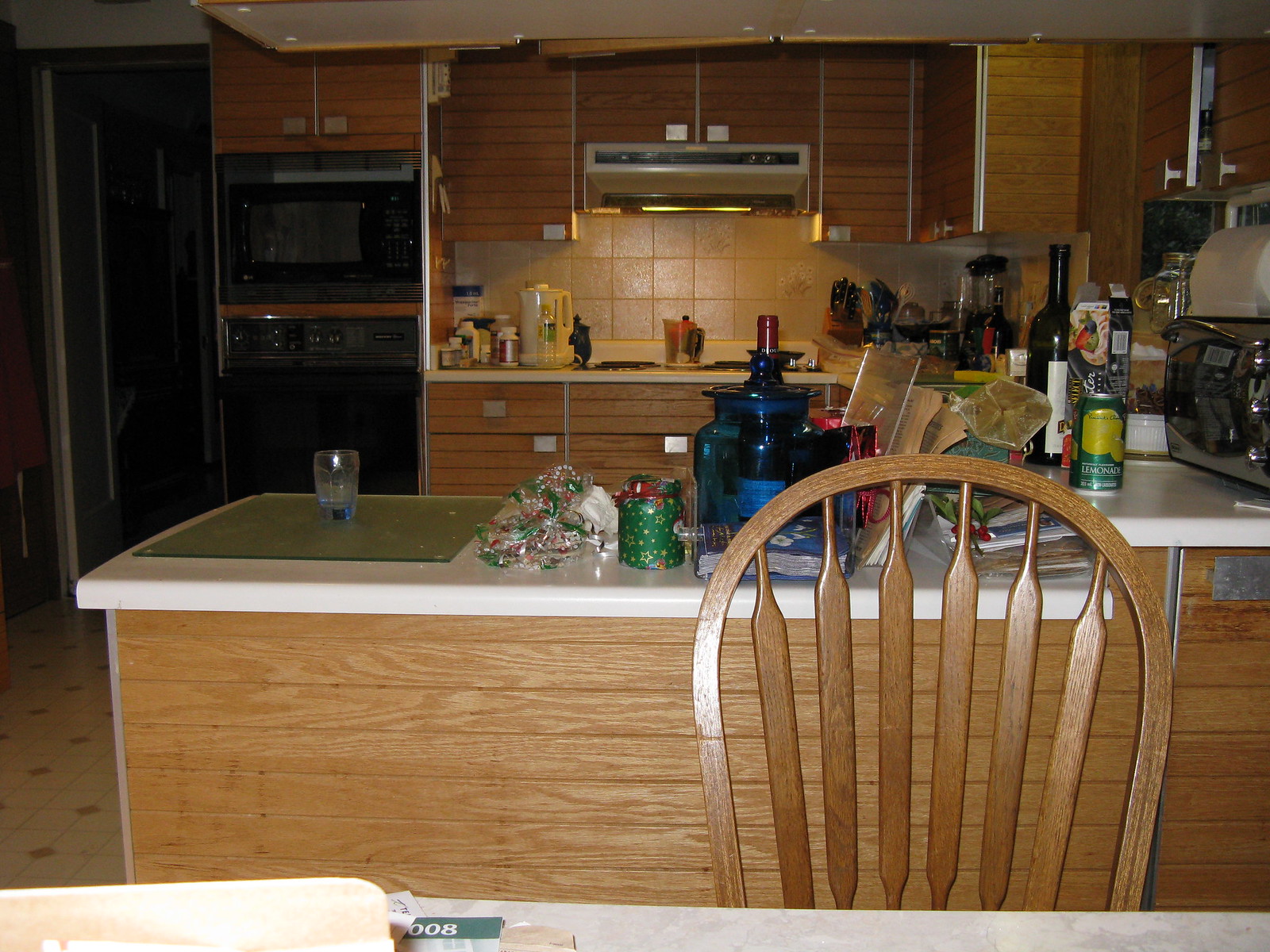The photograph captures the interior of a kitchen, beginning with a dining room chair in the foreground near the edge of a dining table. Moving deeper into the scene, a bar section of the counter is visible, featuring pristine white countertops paired with elegant wooden cabinets. Stainless steel and black appliances are seamlessly integrated into the design, adding a modern touch. To the left behind the bar area, there is a microwave installed above an oven, showcasing efficient use of space. In the foreground, a green cutting board with a glass placed on top can be seen. At the left end of the counter, there is a collection of items, including a bag, several jars, and a few books that appear to be cookbooks, hinting at the kitchen's culinary focus.